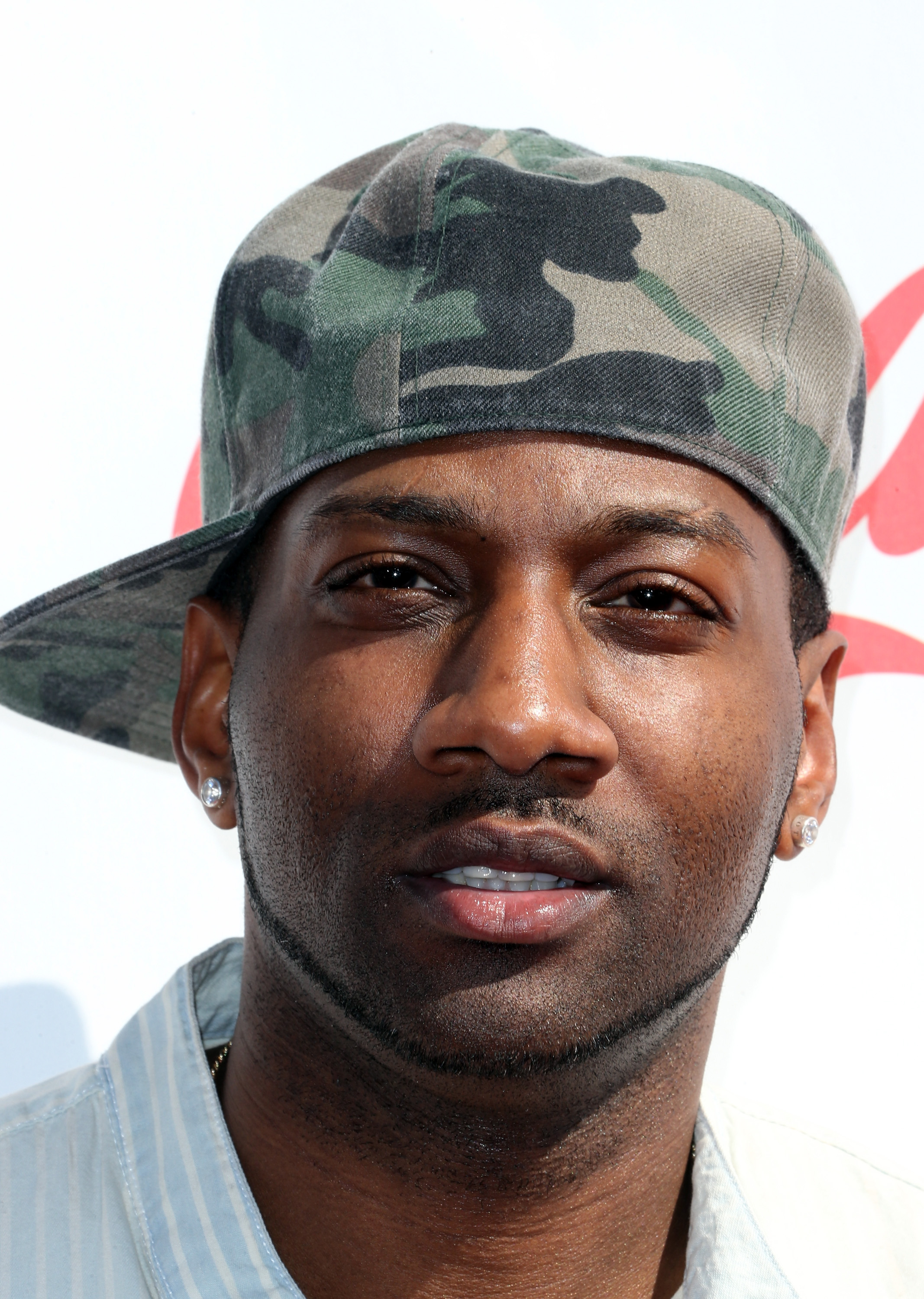The photograph is an outdoor, close-up image taken during the daytime, featuring an African-American male who occupies the center of the frame. He is wearing an army camouflage-patterned baseball cap that is tilted sideways and slightly backward, sitting between his ear and the back of his neck. His facial hair consists of very short, trimmed stubble with a noticeable five o'clock shadow, a thin mustache, and a narrow beard extending just below his chin from ear to ear. The man has diamond stud earrings in both ears and is dressed in a light blue and white collared, button-down shirt. Partially visible is a chain necklace resting around his neck. His eyes are slightly squinted, hinting at bright outdoor lighting. The background is predominantly white with some red writing obscured by his head, likely part of a logo or text, which remains indecipherable. The colors present in the image include red, white, green, black, brown, tan, silver, and light blue.